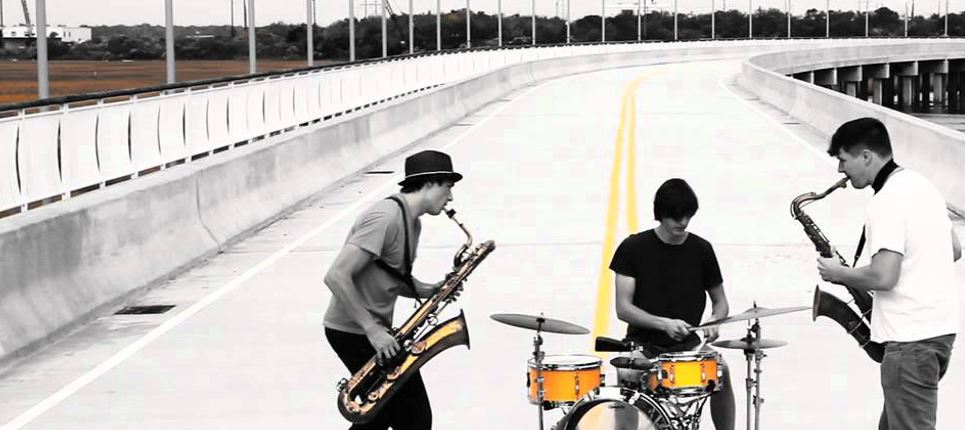The image depicts a surreal scene of three young musicians superimposed on a black-and-white highway, which curves around a bend to the right and features double yellow lines down its middle. The setting appears to be an overpass or on-ramp, made of white concrete with protective barrier walls and white posts spaced evenly in the background. Each musician appears in black and white, except for their instruments and some details, which are in color. 

To the left, a young man wearing a gray t-shirt and a black bowler hat plays a golden saxophone. In the center, another young man in a black t-shirt with shaggy dark hair plays an orange drum set with gray cymbals. On the right, a third young man in a white t-shirt, also with dark hair, plays a saxophone that appears darker in color. The overall image combines elements of reality and digital manipulation, creating a whimsical and intriguing composition.